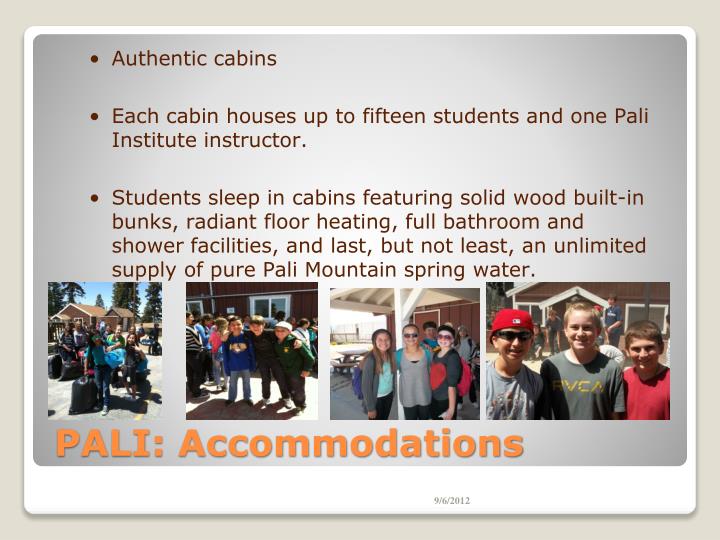The image is a detailed PowerPoint slide advertising Pali Accommodations, with a gray-hued background framed by a white outline. The content is structured with three bullet points in a burnt reddish color on the gray background. The first bullet point highlights "Authentic Cabins." The second point details that "Each cabin houses up to 15 students and one Pali Institute instructor." The third bullet elaborates on the cabin amenities, stating "Students sleep in cabins featuring solid wood built-in bunks, radiant floor heating, full bathroom and shower facilities, and an unlimited supply of pure Pali Mountain spring water." Below these points, the slide features four photos showing numerous happy and smiling campers posing in front of cabins. At the bottom of the gray slide, in large orange letters, it says "Pali: Accommodations." Below the entire slide, a white background displays the date "9-6-2012" in small letters.